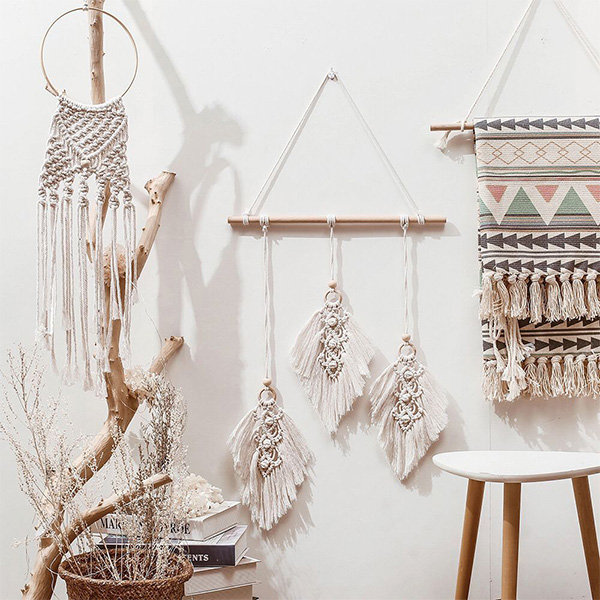This close-up, realistic photograph showcases a series of Navajo-style wall hangings arranged against a white background. On the left, a slim, round, whitewashed tree branch leans against the wall, adorned with a round wooden circle from which a dreamcatcher with intricate weavings and tassels dangles. Resting beside this branch is a basket filled with whitewashed bare tree branches, accompanied by a stack of white and black books. 

In the center of the composition, a large dreamcatcher featuring three tasseled segments hangs from a white nail. The centerpiece is suspended by twine forming a triangular support structure. 

To the right, a Navajo blanket, which has been folded over, displays two rows of tassels and is hung by a white string. Below this on the bottom right, a three-legged stool with a white top can be seen, completing the rustic, yet artful, arrangement. The overall display blends Navajo craftsmanship with decorative, natural elements.